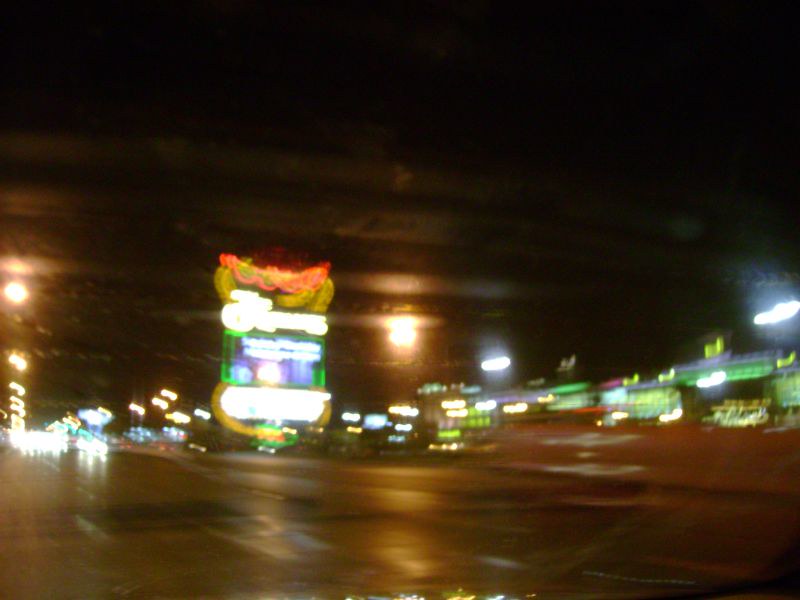A blurry nighttime photograph captures the vibrant energy of a bustling city street. The scene is dominated by an array of large neon signs, particularly one prominent sign glowing in yellow, orange, blue, and white lights on the left side of the street. Traffic fills the wide road, with car lights creating streaks that add movement to the image. Overhead, tall streetlights contribute to the city's illumination. Buildings line the street, their facades adorned with blue rooftops and green-lit windows. The road glistens slightly, suggesting a recent rainfall, and enhancing the multitude of lights that define this urban nightscape.